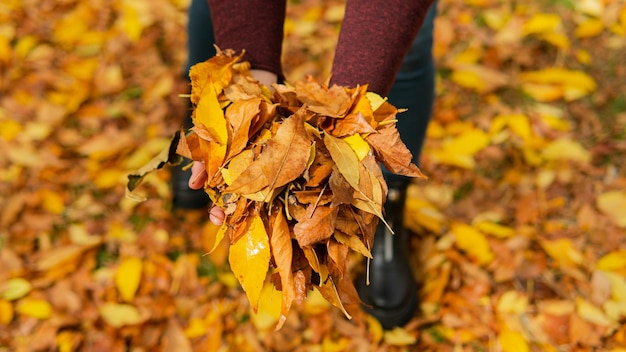In this detailed and vibrant autumn scene, a person wearing a long-sleeve red sweater and black jeans with black boots is holding a bunch of yellow and brown leaves towards the camera. Their forearms are extended downwards, making the colorful leaves the focal point of the image. The ground surrounding them is completely covered in a bed of scattered autumn leaves, adding to the rich tapestry of yellows, browns, and oranges characteristic of the season. The backdrop is blurred, drawing sharp attention to the hands and leaves, all captured with impressive clarity, leaving no visible signs of grass or other background elements. This close-up, taken in crisp detail, emphasizes the lush and vibrant nature of fall.